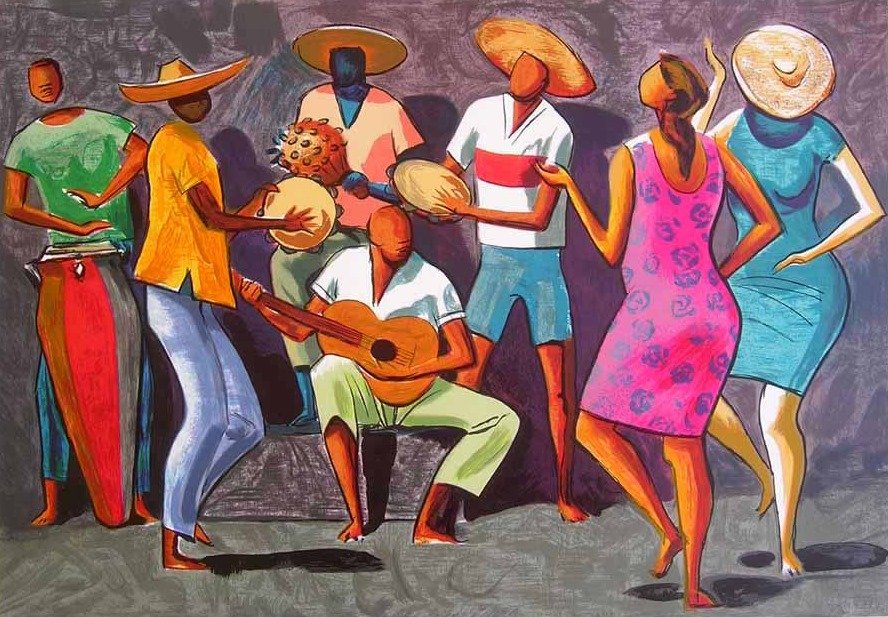This animated image depicts an animated, colorful scene of seven people celebrating and dancing together. On the left, a lively band of five musicians delivers a festive atmosphere. The band features a seated guitarist in green pants and no shoes, a man in a green shirt playing a large red drum with his hands, and three standing members wearing wide-brimmed sombrero hats. Two of these hat-wearing musicians enthusiastically play tambourines, while another, with bluish skin, shakes a large maraca. Each band member is clothed in vibrant attire, adding to the image's rich palette.

To the right of the band, two women in dresses dance joyfully to the music. One wears a pink dress adorned with purple flowers, while the other dons a teal dress. Despite the lively actions and colorful clothing, the characters' facial features are mostly blank, emphasizing their motions and interactions rather than their individual expressions. The background of the image is gray, providing a neutral backdrop that highlights the festive and colorful foreground. This cartoonish and meticulously detailed image perfectly captures the spirit and energy of a jubilant celebration.